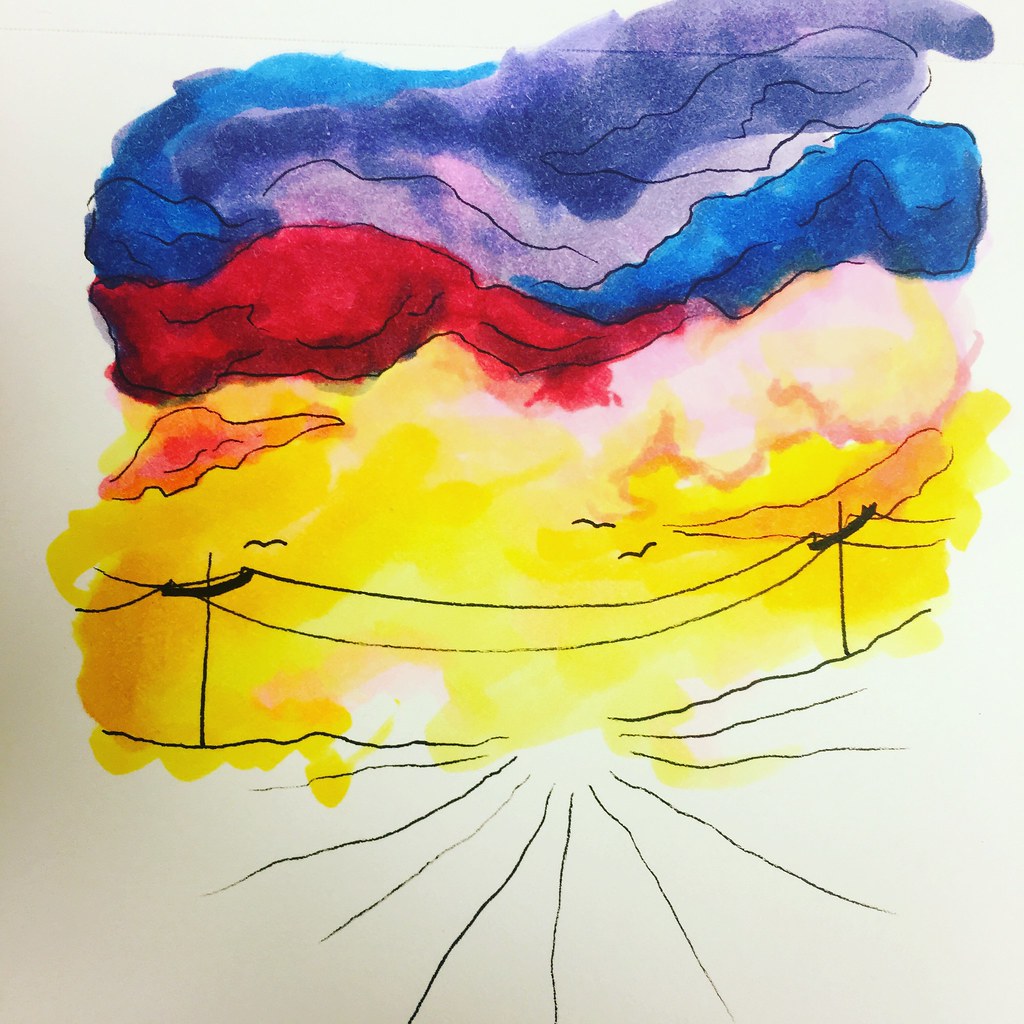This image is a vibrant, loosely painted night sky on an off-white, slightly gray-toned background towards the lower left corner. In the center, a splotchy yellow base transitions into an array of colors, mimicking a sunset. From a wavy-lined road, black ink power lines stretch across, suspending between telephone poles. The sky, accented by pink, red, blue, and purple clouds, features three simplistic birds shaped like upside-down Ws. The gradient sky begins with a bright yellow at the bottom, blending into reds, blues, and purples, with the clouds becoming darker as they reach the top. This dynamic mix of black ink and vibrant watercolors on the white paper gives a dramatic yet serene depiction of an evening sky.